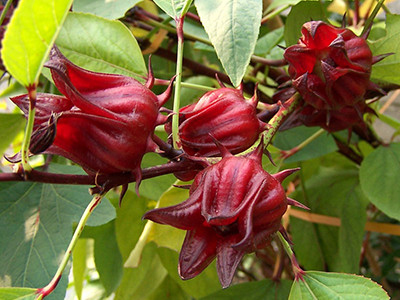This highly detailed, close-up photograph captures four deep burgundy flowers on a vine, surrounded by abundant green leaves. The flowers, which strongly resemble either partially opened roses or tulips, exhibit a rich, dark red color and a waxy, almost rubbery texture. Sunlight filters through the leaves, casting interesting shadows and making some leaves appear lighter and nearly translucent. The flowers are not fully open, with their petal tips beginning to part slightly like the opening mouth of a flower, and spikes or thorns are visible at their bases. Some stems are noticeably reddish while others are green and brown, enhancing the natural, outdoor setting of this blooming plant.